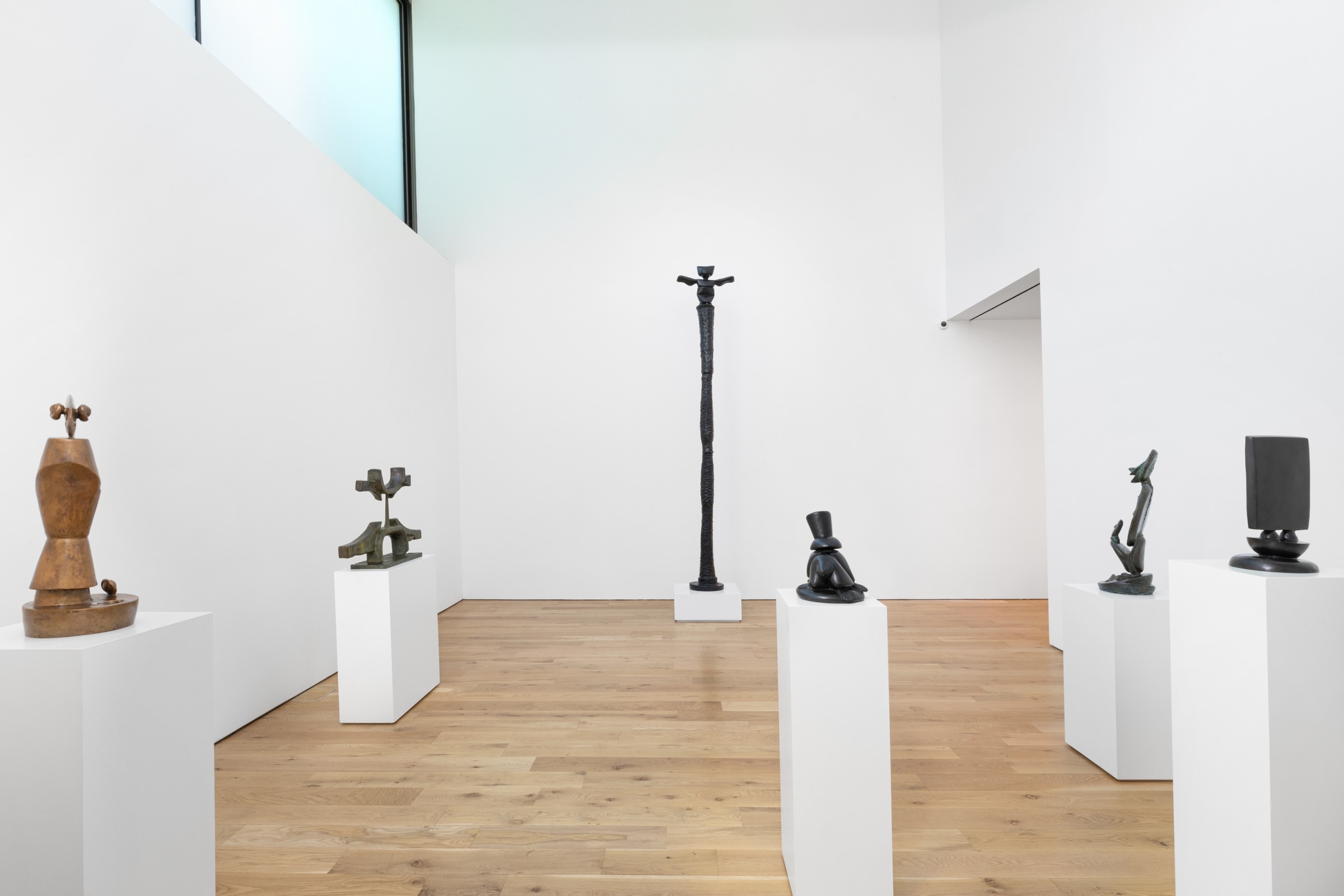This image showcases the interior of a pristine art gallery or museum room with minimalistic design. The room features white walls and high ceilings, with a large window situated in the top left corner that brings in natural light. The flooring is made up of light-colored hardwood, adding to the airy and polished atmosphere. 

In terms of displays, there are six pedestals arranged throughout the room, each holding sculptures. Five of these pedestals are taller and predominantly black, each supporting a shorter, abstract statue. A notable exception is a shorter white pedestal that supports a strikingly tall and totem-like sculpture, which stands out due to its height. Among the statues, all are black except for one, which appears to be carved from a brownish wood and is situated on the left.

Additionally, a doorway or entryway is present on the right side of the image, suggesting a passage to another part of the gallery. The overall scene is calm and devoid of people, allowing the focus to be solely on the art pieces and the room's minimalist, yet elegant design.